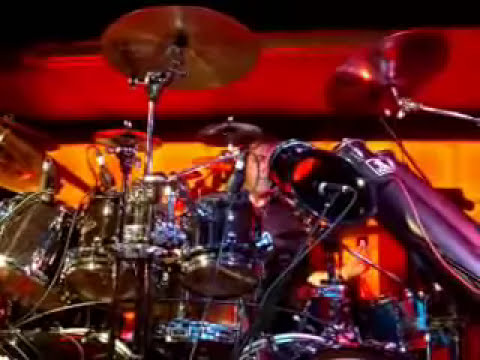The wide rectangular image captures a detailed, professional-grade drum set on a dimly lit stage, prominently situated on the left side. The drum set consists of numerous cylindrical drums with black metallic bands around them and silver metal bottoms. A maze of silver poles supports various cymbals, including one descending from the top right corner. Amidst the drums, a white male drummer with dark brown hair and a black shirt is partially visible, hinting at his central role in the performance.

Behind the drummer, the background features a stark contrast of glowing lights: a horizontal neon red light at the top, a dark band below it, followed by a brightly lit orange section. The vibrant colors—red, orange, gold, silver, blue, purple, and pink—enhance the concert atmosphere, while wires intricately lace the drum kit, each drum head meticulously miked for optimal sound recording. The overall scene suggests a high-energy live concert performance, emphasizing the complex and sophisticated setup of the drums under dramatic lighting.